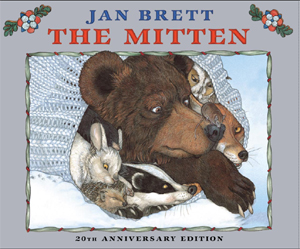This image features the front cover of the 20th Anniversary Edition of the picture book "The Mitten" by Jan Brett. Set against a gray rectangular background, the top of the cover displays "Jan Brett" in blue text, while the title "The Mitten" appears prominently in larger red text. At the bottom, "20th Anniversary Edition" is written in black text. The top corners of the cover are adorned with festive, Christmas-like decorations in green, red, white, and blue, resembling little banners.

The central illustration, enclosed by a border decorated with green outline and red beads, depicts a cozy, snowy scene. A large white mitten holds a collection of animals, each peeking out adorably. The bear, the largest of the animals, is centrally positioned, with part of its head and hand visible. To the left, a rabbit, hedgehog, and skunk share the cozy space, while to the right, an owl and fox crowd in. The mitten's pocket also reveals a white bunny, an orange fox, a black and white opossum, and two other creatures, all set against a blue background. This picturesque composition conveys a warm, wintry feel, echoing a Christmas theme with two mistletoe decorations positioned at the top left and top right of the cover.